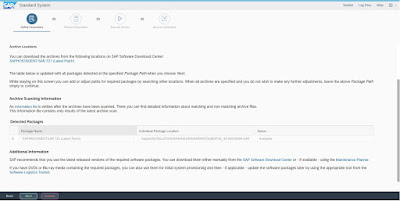The image is a small, horizontal rectangle with text that is difficult to read due to its size. The top edge features a turquoise line running horizontally from left to right. Just beneath this line, there is a logo situated in the upper left corner, accompanied by some unreadable text to its right. The background behind this text and logo is light gray. The upper right corner also contains some text.

As you look further down, the background turns white. The first noticeable element is text highlighted in blue. Below this, there are various icons that are not clearly visible. This is followed by two lines of black text, succeeded by some turquoise text, and then some more black text. There is a bold black heading with additional text beneath it. Following this heading are three light gray fields designed for input, each presumably allowing for some form of data entry.

Towards the bottom, there's another section of bold black text with additional text underneath it. Finally, at the very bottom of the image, there is a horizontal black rectangular area containing small icons on the left-hand side.